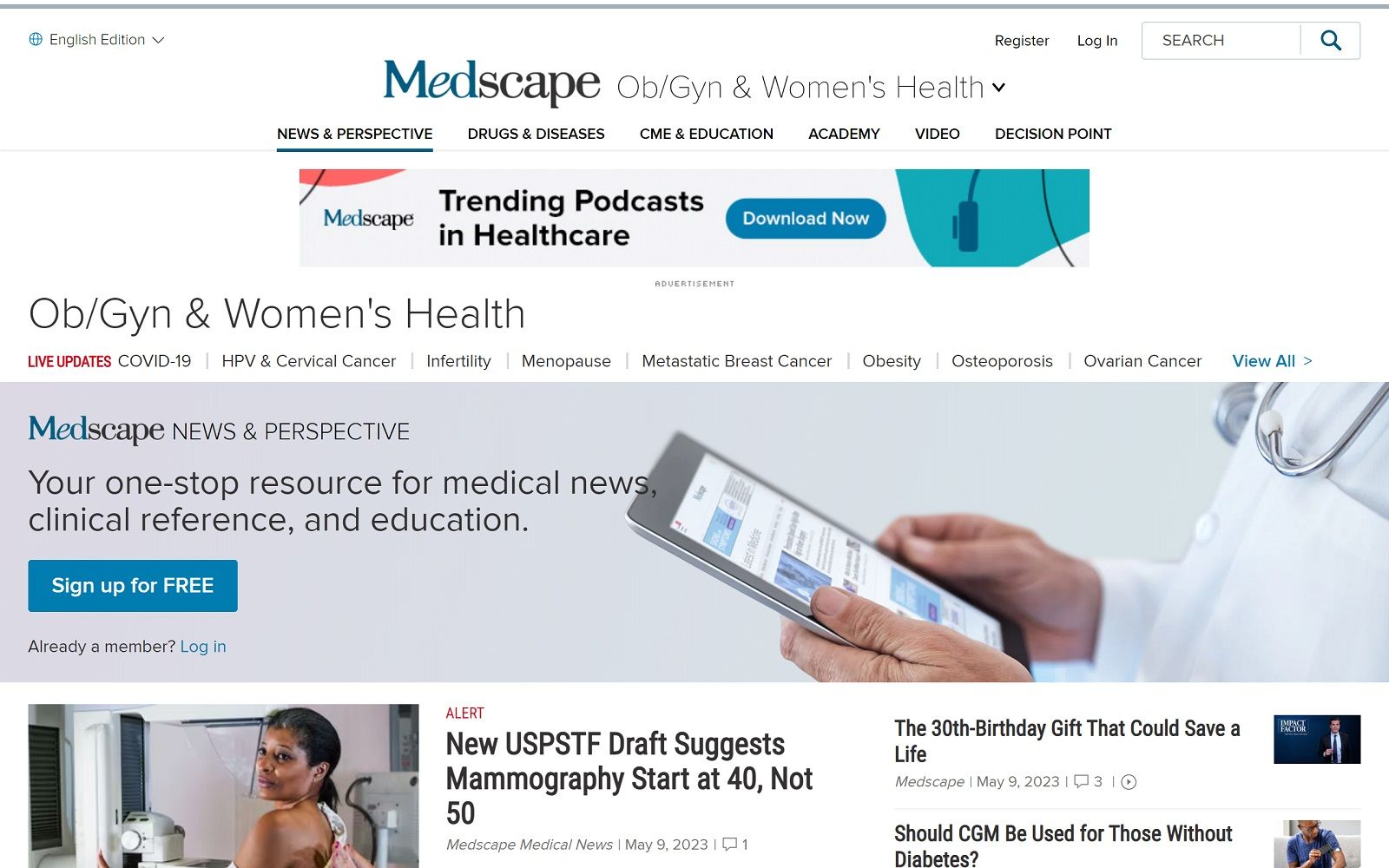Screenshot of the Medscape homepage and navigation options, featuring a blend of informational categories and interactive elements. The page includes links for registration and login at the top, followed by a prominently placed search bar. Featured sections include areas for news, respected articles on drugs and diseases, CME and education opportunities, an academy, videos, decision points, and trending healthcare podcasts. Medscape's mobile app is also promoted with options to download. Live updates cover a variety of health topics like COVID-19, cervical cancer, infertility, endopathy, metastatic breast cancer, obesity, osteoporosis, and ovarian cancer. The page is designed to coordinate numerous resources, highlighting Medscape’s offerings under repeated headings like "lb/jyn," "womentel," and other key anchors.